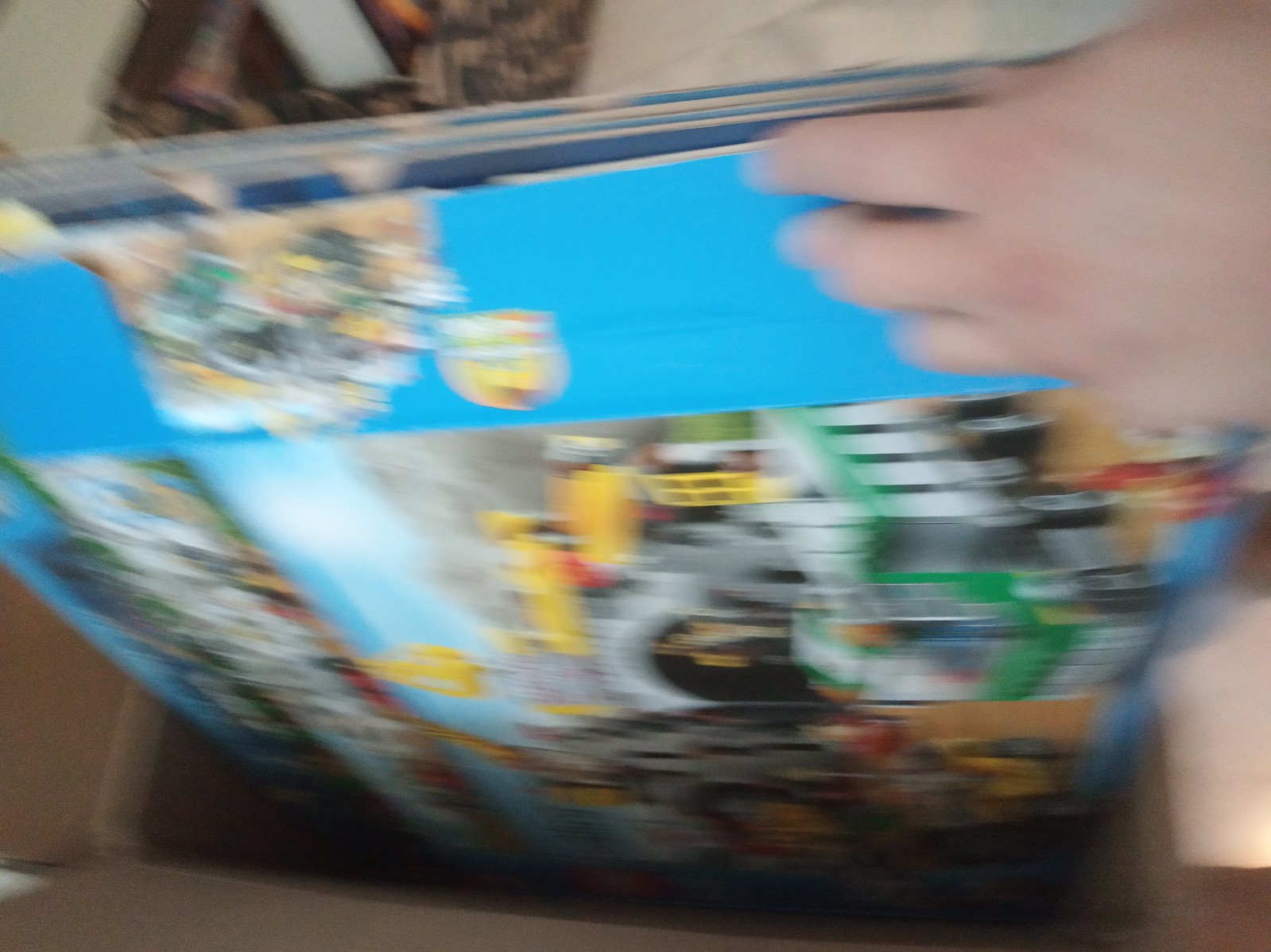In this somewhat blurry image, the focal point is a large cardboard box from which people appear to be pulling out smaller, folded cardboard boxes. These smaller boxes are predominantly blue and darker blue in color and seem to be neatly packed inside the larger one, possibly for display purposes. A hand, emerging from the top right corner, obscures part of the view; the thumb is out of frame, but the rest of the fingers are visible. The floor is tiled in a tan color, while in the background, there are indistinct brown and black objects partially cut off by the image's edge. The contents inside the boxes suggest they might be related to a Lego set, given the visible green and white truck and some yellow elements, although the blurriness of the image makes it difficult to precisely identify the set.